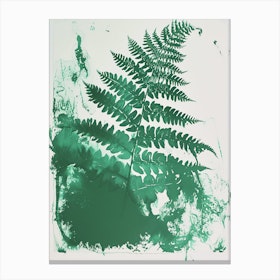The image depicts a tall, slender stem of a fern illustrated on an off-white canvas. The fern, which displays fractal characteristics, has leaves that emanate symmetrically from the center, starting wide at the base and tapering to narrow tips towards the top, resembling the shape of a Christmas tree. Painted primarily in varying shades of green, including a prominent dark green blotch in the lower left corner, the watercolor artwork uses a consistent green color palette. The fern's detailed leaves and slender branches intricately spread out along the stem, creating a natural and delicate appearance against the plain white background. Additional green splatters adorn the lower and upper portions of the canvas, adding a touch of abstract expression to the artwork.